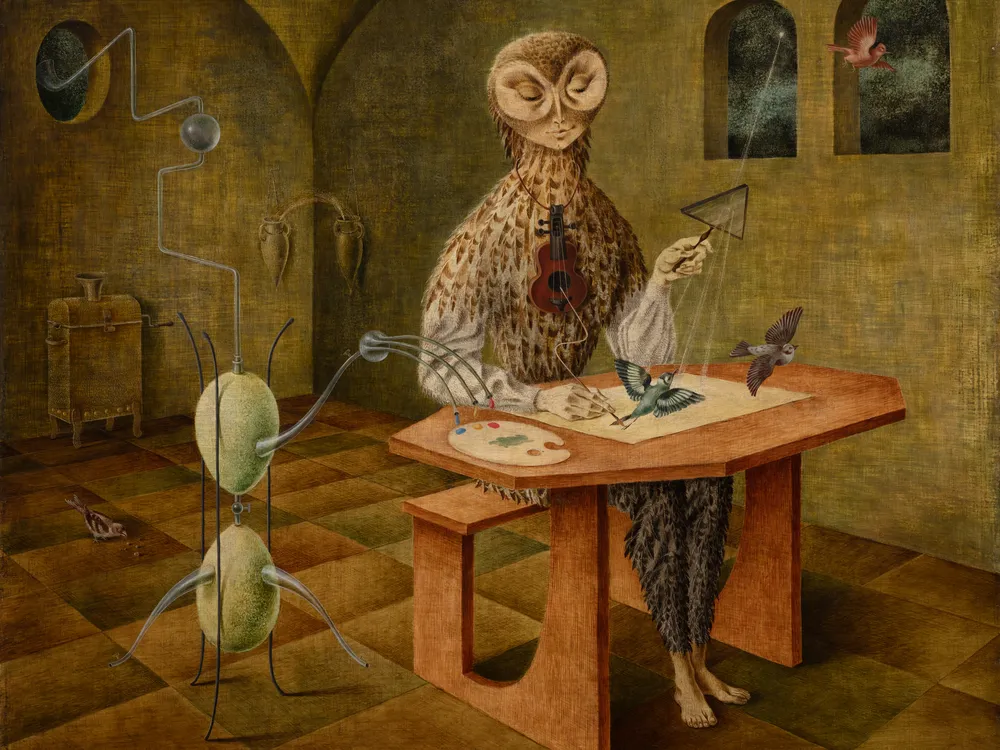The artwork in question is an intriguing and abstract painting characterized by earthy tones. Set within a room with green concrete walls and a wooden-tiled floor, a peculiar scene unfolds. At the center sits a hybrid creature, part human and part owl. This owl-human figure features an owl’s head with feathers descending down its neck and body, juxtaposed with human arms and legs, which are also adorned in feathers. The creature is seated at a wooden school-like desk, intensely focused on its artistic endeavor. Around its neck dangles a necklace with a miniature violin, adding an enigmatic touch.

The creature is deeply immersed in its craft, using its right hand to draw a pair of birds on a piece of paper, seemingly bringing them to life. The birds, which appear blue and purple, lift from the page in a vibrant, three-dimensional effect. A red bird can be seen higher up, near a window. In its left hand, the owl-human holds a magnifying glass shaped like a triangle, emitting beams that animate the sketch.

Adding to the strangeness of the scene is an adjacent peculiar contraption—a tubing system that appears to provide paint from outside the room. This paint is funneled into a two-headed alien-like creature with grape-shaped features. The paint, colored blue, yellow, and red, is then mixed into the owl-human's drawing instruments, accentuating the surreal and otherworldly nature of the artwork. Birds fly around, enhancing the life-giving energy that permeates this curious and imaginative piece.